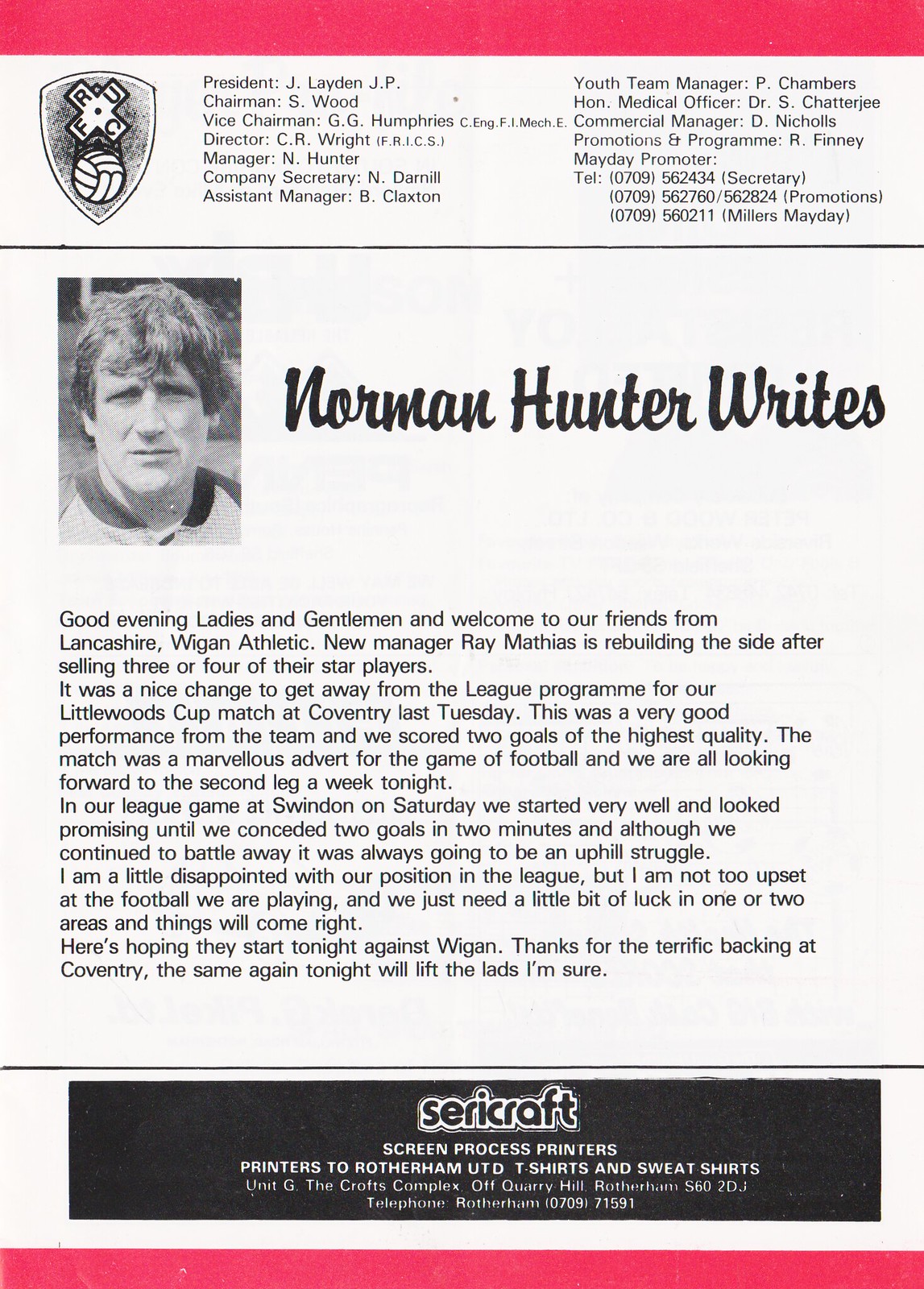This predominantly black and white print piece, bordered by a striking red line at the top and bottom, appears to be a detailed newsletter likely from a sports team magazine dedicated to soccer. The upper two-thirds of the page feature a photograph of a man accompanied by the text "Norman Hunter Writes." Next to the image, it states, "Good evening ladies and gentlemen, and welcome to our friends from Lancashire." It outlines how the newly appointed Wigan Athletic manager, Ray Mathias, is in the process of rebuilding the team after parting ways with several star players.

To the left, there is a shield-shaped team logo in black and white, featuring a soccer ball and a tilted cross. The central text comprises a welcoming message and a report on recent matches, including highlights from a thrilling Little Woods Cup match at Coventry where the team scored impressive goals, and a challenging league game at Swindon. Despite setbacks, there is a hopeful tone about the team's future performance.

The bottom of the page lists key organizational figures, such as the president, chairman, vice chairman, director, and managers, including the youth team manager. It also features multiple contact numbers for these personnel. Highlighting the professional craftsmanship, the document credits 'Sarah Craft Screen Process Printers,' noted as the printers for Rotherbay UTD’s t-shirts and sweatshirts, suggesting a dedicated effort towards team branding and community engagement.